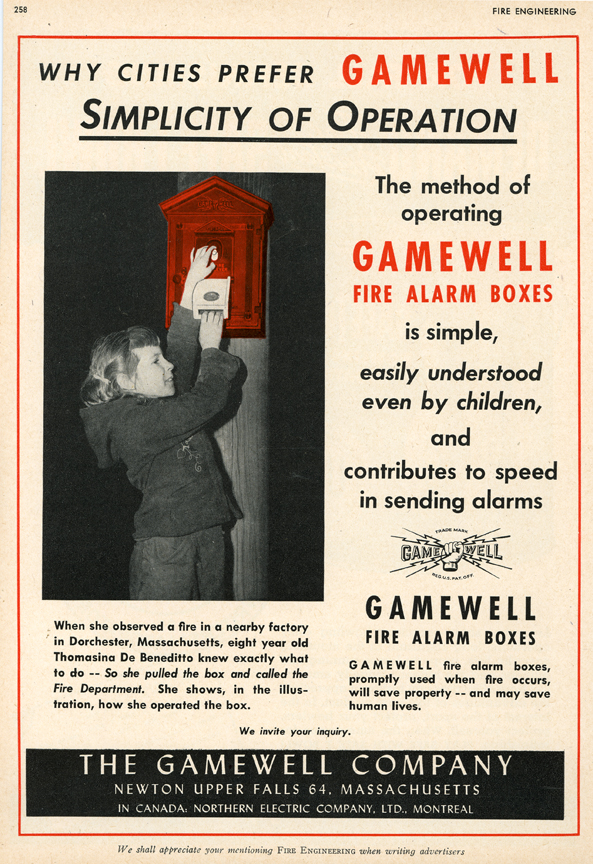This is an advertisement poster featuring a black-and-white illustration of a child demonstrating the simplicity of operating a GameWell fire alarm box. The image, centrally placed on the left-hand side, depicts an eight-year-old girl named Tomasia DiBendito confidently pulling a lever from a red fire alarm box mounted on a pole, while wearing dark-colored clothing and smiling—a testament to the device's ease of use. The textual content of the poster emphasizes the practical and life-saving benefits of GameWell fire alarm boxes, highlighting the company's claim: "Why cities prefer GameWell - simplicity of operation." It explains that the method is so straightforward that even children can understand and quickly operate it, thereby enhancing the speed of sending alarms. The poster also mentions that the advertisement is from the GameWell Company located in Newton Upper Falls, Massachusetts, with a Canadian branch in Montreal operated by Northern Electric Company Limited.